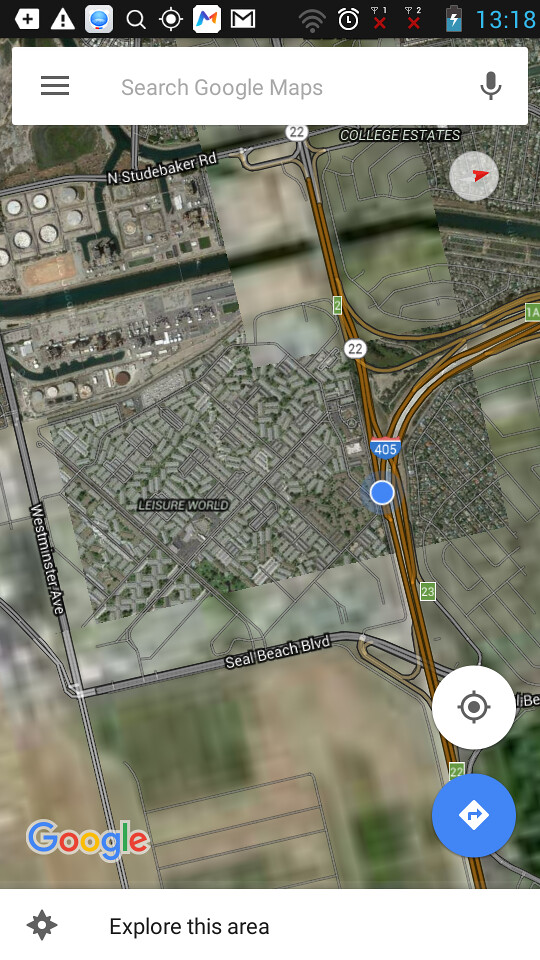This Google Maps image displays a detailed navigation screen from a smartphone. At the very top, a status bar includes various icons such as an email symbol situated towards the right, network signal indicators, an alarm clock, two red "X" marks, and the number 1318 in the upper right corner. Directly below this, a rectangular search bar labeled "Search Google Maps" is visible. This bar features a hamburger menu icon on the left and a microphone icon on the right for voice search functionality.

The main content of the image reveals a map focusing on a freeway, identified as Route 405, which curves prominently to the right along the right edge of the map. A blue dot just below the freeway marker indicates the user's current location. To the left side of the map, two labeled streets intersect: Seal Beach Boulevard, stretching to the left, and Washington Avenue, running perpendicular to it.

In the bottom left corner of the map, a small "Google" branding is present, and at the very bottom of the image, outside the map boundary, the prompt "Explore This Area" invites further interaction.